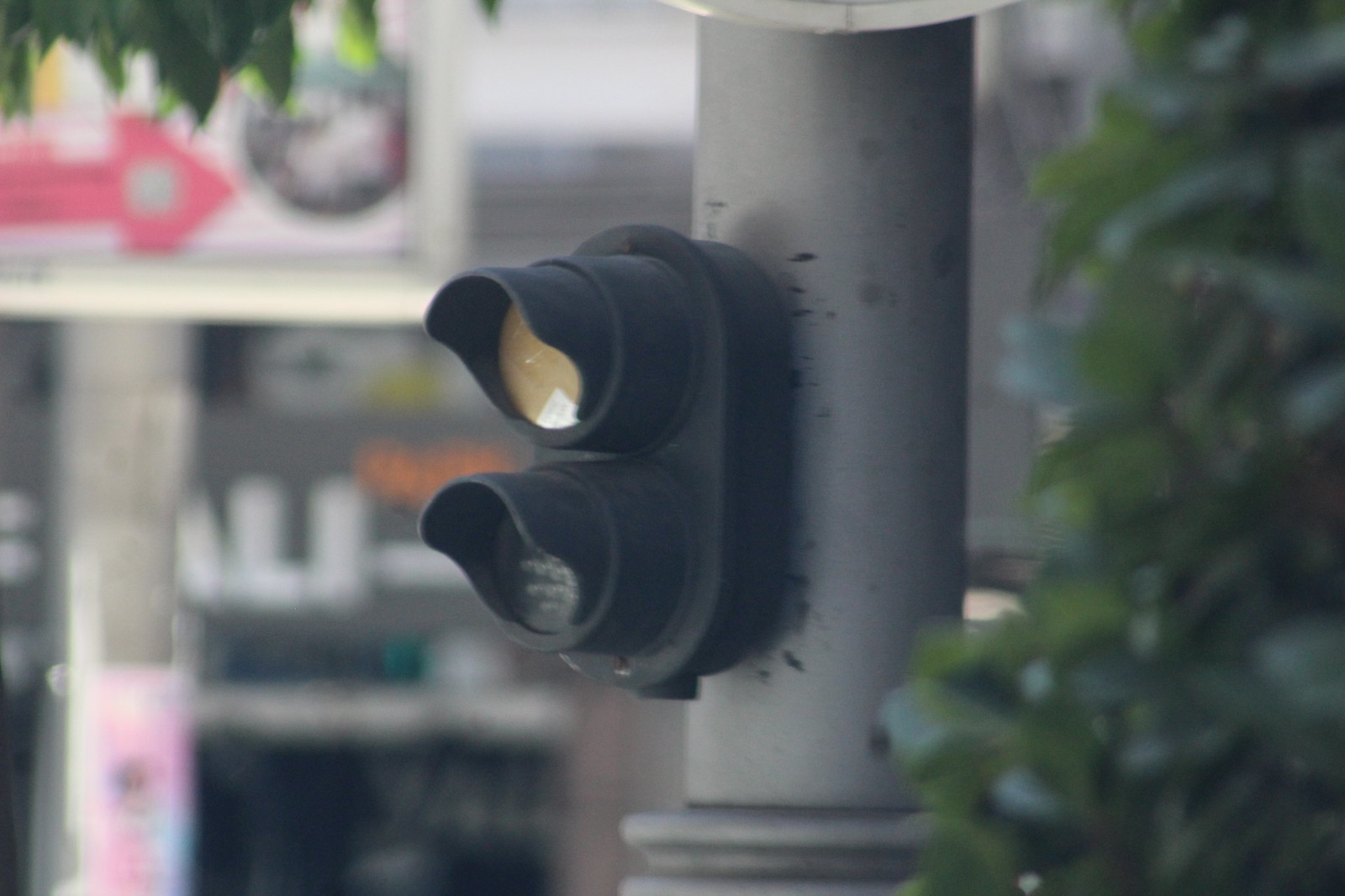The photograph captures a close-up of a gray, cylindrical street pole with a black, oval-shaped traffic light attached. The traffic light features two circular lights: the top one is yellow, and the bottom one appears gray, as it is not illuminated. Dominating the right side of the image is a large, dark green bush with oval leaves, and similar green vegetation is mirrored in the top left corner, giving the impression that the photo might have been taken from within the bushes. The background is intentionally blurred highlighting the foreground elements; however, a billboard with a bright red arrow and a central square is faintly visible in the top left, adding depth to the urban setting. The composition suggests a potential stop-and-go function for the traffic light, but its exact purpose remains ambiguous due to the absence of any active light signals.